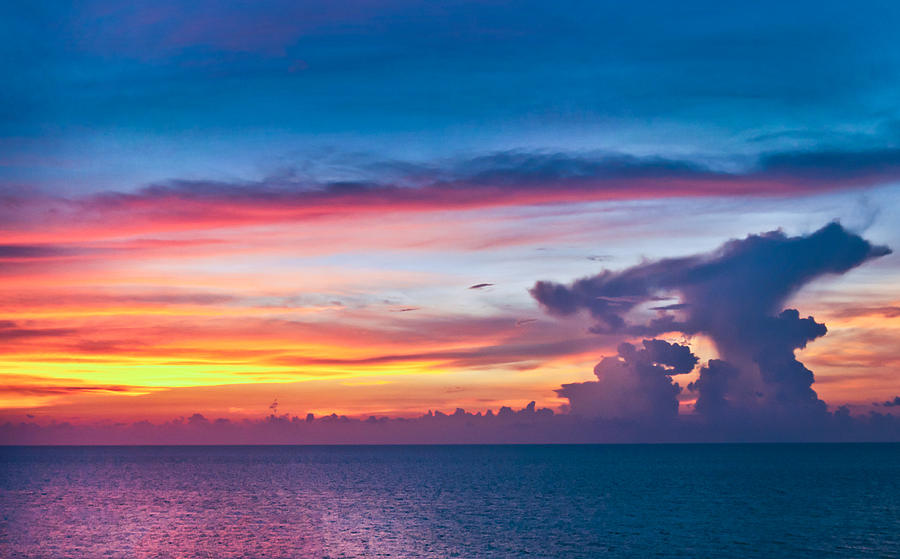The photograph captures a mesmerizing ocean sunset with a dramatic and colorful sky. The calm ocean stretches across the bottom of the image, displaying a few gentle ripples. The horizon glows with vibrant yellows and oranges, blending into the blue tones of the evening sky. In the middle right portion of the photograph, towering clouds rise dramatically, almost resembling explosions, with one larger and more pronounced than the other. These clouds contain hues of dark navy blue and pink, creating an impression of flames against the backdrop of the sky. The entire scene presents a breathtaking dance of colors, with layers of clouds that appear to be ignited by the sunset, adding a fiery ambiance. The shoreline and some distant trees can be faintly seen, grounding the scene in a serene and picturesque setting.